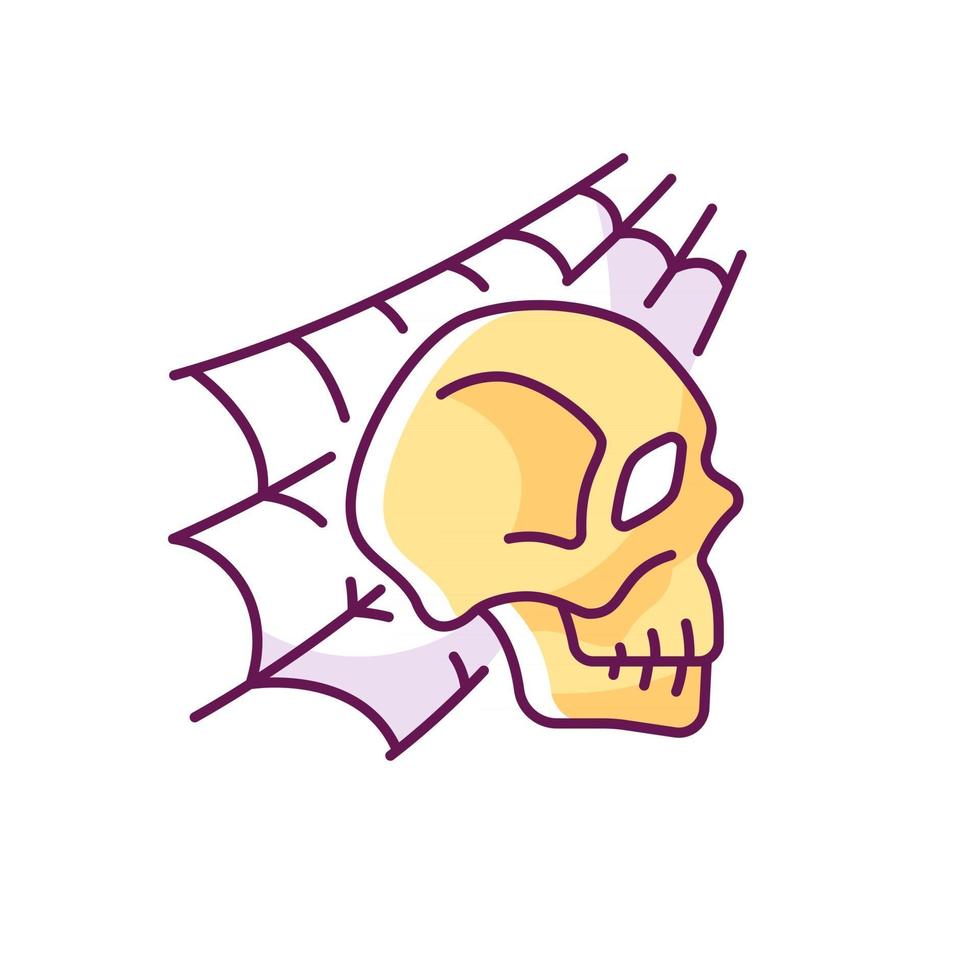In this image, a digitally drawn, cartoonish skull is positioned on a completely white background. The skull, rendered in shades of light yellow, light orange, and off-white, is facing to the right, revealing its right side along with empty eye sockets and the nasal cavity. Overlaying the skull, particularly on its top right, is a simply drawn purple cobweb, whose strands stretch from the bottom left to the upper right of the image. This cobweb consists of multiple intersecting lines, structured as columns and rows, giving it a lightweight and somewhat whimsical appearance. The overall aesthetic of the image leans towards a gothic or horror-inspired cartoon style.